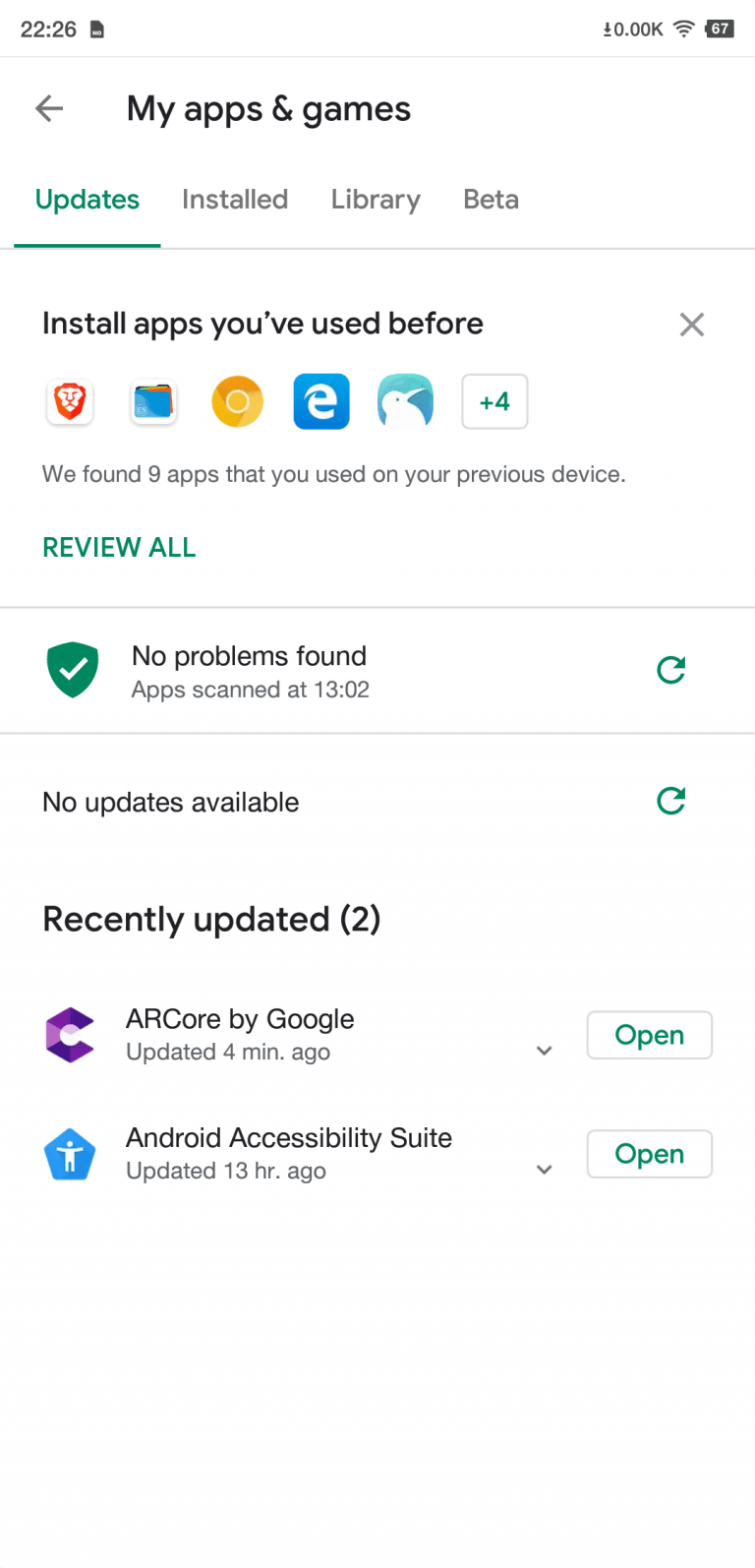The screenshot is an overview of various app categories on a device. The interface header reads "My Apps and Games," and it is organized into several sections: "Updates," "Install," "Library," and "Beta." A prompt encourages users to re-install previously used apps, displaying several unfamiliar app icons. There is an option to "Review All" with a status message stating "No Problems Found" and "Apps Scanned at 1302." Further details indicate "No Updates Available" and show recently updated apps, listing "ARCore by Google" and "Android Accessibility Suite," marked with a numeral "2."